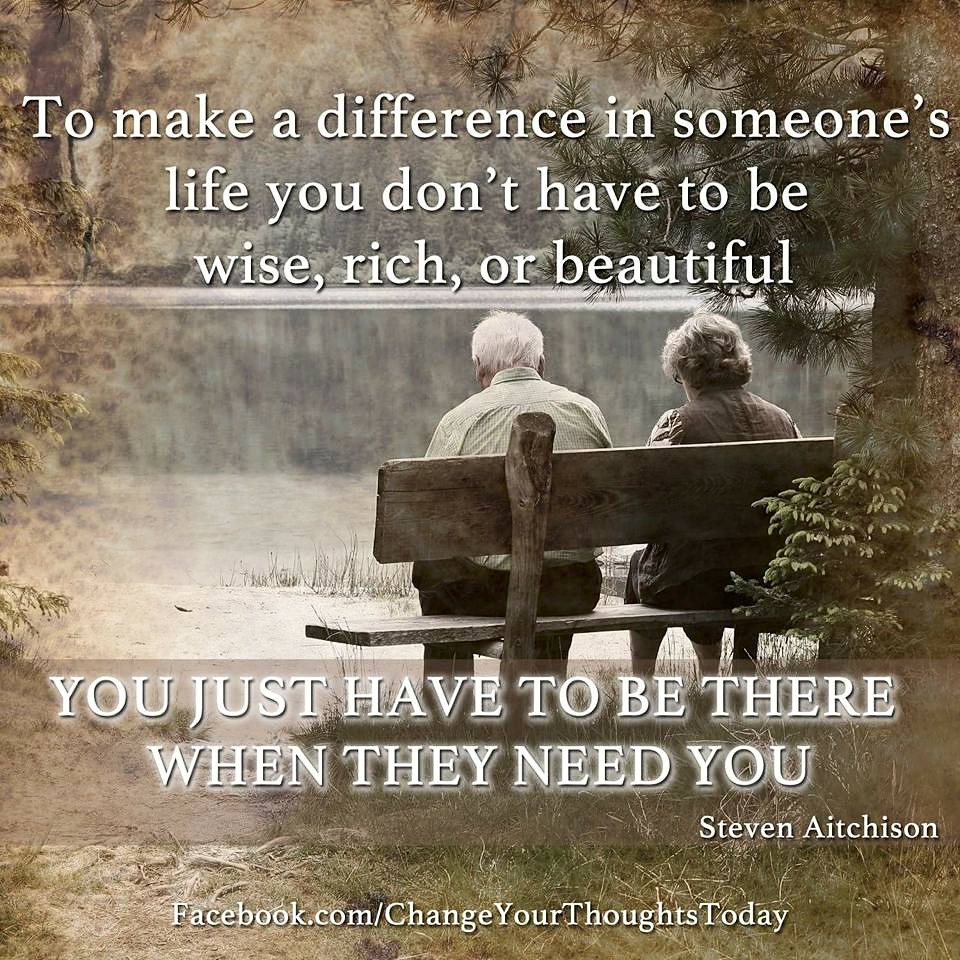The image is a well-framed poster featuring a serene photograph of an elderly couple, known as the Bats of Tuesta, seated on a wooden plank bench. The couple, an older man with white hair wearing a light shirt and dark pants and a woman with grayish hair dressed in a light purple dress, are facing a small lake or pond surrounded by light green shrubbery. A pine tree is evident behind them, with its needles appearing just above their heads, and the calm water reflects the trees. 

Above the couple, a heartwarming quote in white lettering reads, "To make a difference in someone's life, you don't have to be wise, rich, or beautiful." Beneath the bench, additional text declares, "You just have to be there when they need you." The quote is attributed to Stephen Atchison. At the very bottom of the poster, in white letters, the URL "facebook.com/changeyourthoughtstoday" is displayed.